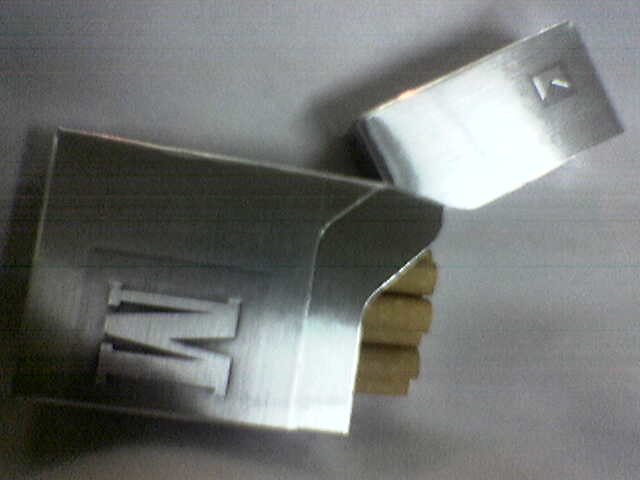The photograph is a slightly fuzzy, rectangular image of a partially open silver cigarette pack resting on a table or counter. The packaging resembles brushed aluminum, with an embossed capital "M" on the front, suggestive of the Marlboro logo. The pack opens uniquely, akin to a Zippo lighter, with a hinged lid that pops open and to the side. Inside the pack, about five to six cigarettes are visible, their brown filters sticking out. The overall image is somewhat out of focus, possibly taken with an older camera, and features a white-gray background with subtle shadows. The shiny, metallic surface of the box stands out prominently against this muted backdrop.